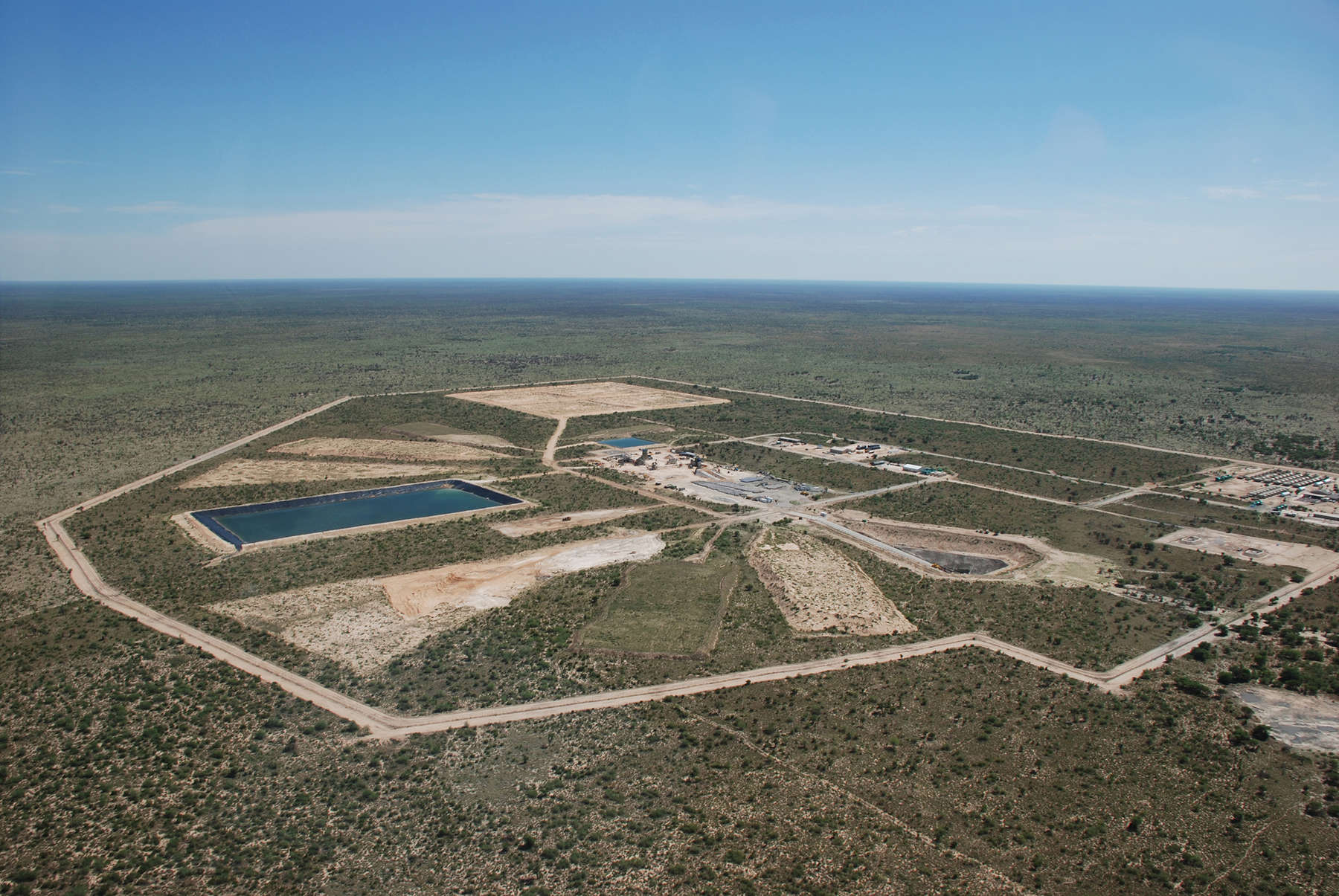This is an aerial image, taken from a very high altitude, giving us a wide view of the landscape below. The central focus is a meandering road that starts at the bottom right corner and twists diagonally across the image, creating multiple sharp zig-zag turns, which eventually extend towards the upper left before angling back to the right and slightly downward, suggesting it might reconnect with the starting point off-frame. The terrain appears arid and barren, dominated by brush land with sparse vegetation and scattered small trees. There are numerous dirt paths crisscrossing the area, and within these paths, a few structural features stand out.

Near the central road, there's a notable enclosed area that contains a rectangular pool lined with black plastic, possibly for water storage, mining, or some industrial purpose. Additionally, one corner of this area has a square, light brown patch, resembling either a building or a large piece of equipment. The landscape also includes several lighter and darker brown patches interspersed throughout, suggesting the presence of rock, sand, or other natural materials, as well as small buildings or other industrial structures.

Despite the desolate look of the area, the horizon is visible in the distance, giving a sense of the vast expanse of land. The distant blue sky contrasts with the earthy tones below, reinforcing the sense of a remote and largely uninhabited region.